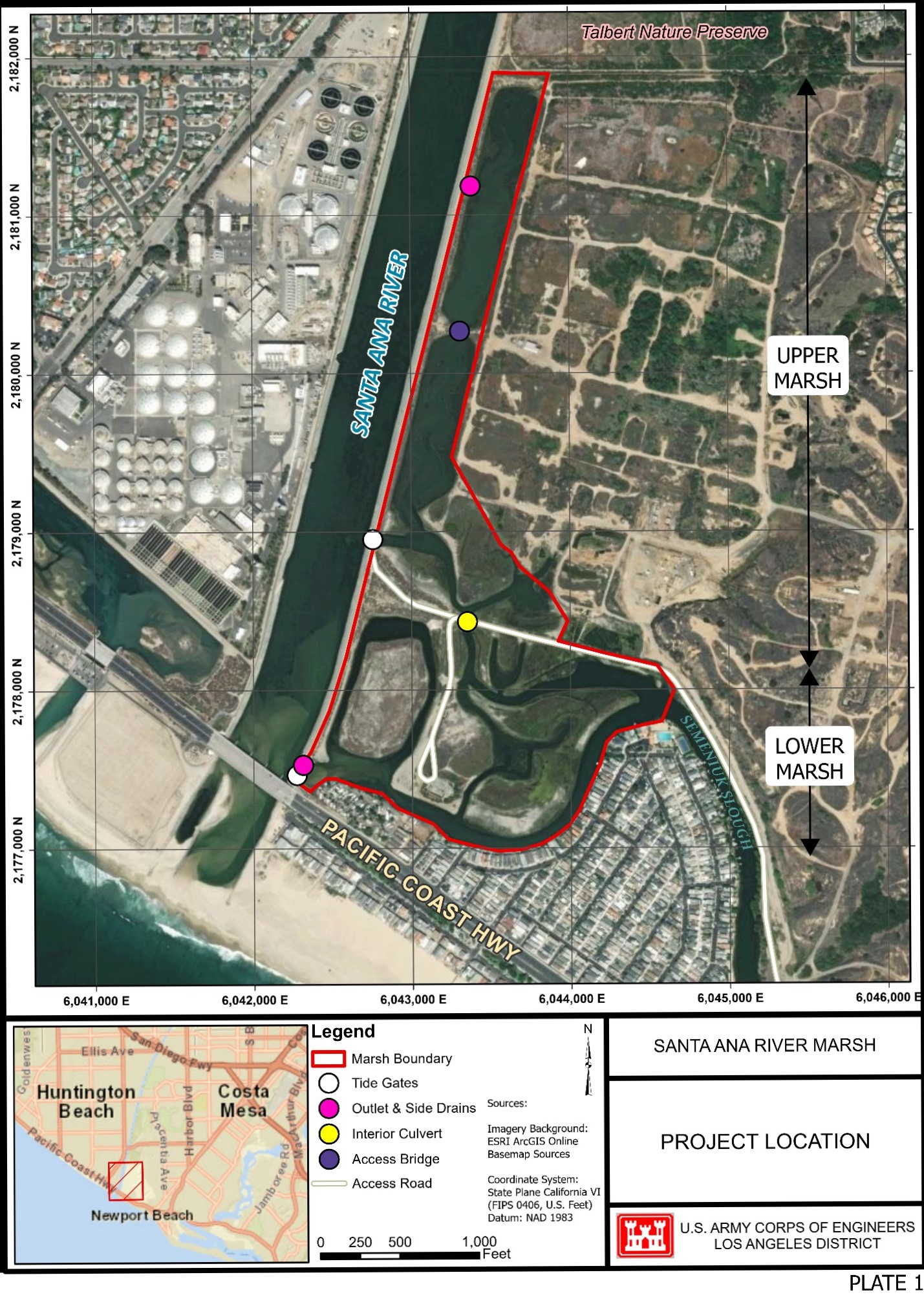This aerial map, titled "Plate 1," is produced by the U.S. Army Corps of Engineers, Los Angeles District. It depicts the project location for the Santa Ana River Marsh, an area situated between Huntington Beach, Costa Mesa, and Newport Beach, along the Pacific Coast Highway. The map is detailed with demarcation lines of the project outlined in red, and highlights the Upper Marsh, Lower Marsh, and the Santa Ana River flowing into the water at the bottom left. Additional features include a scale on the left and a legend with measurements in miles and feet in the middle. A larger inset map at the bottom left corner shows the regional context with cities and the area outlined. The bottom right corner is labeled "Santa Ana River Marsh, project location."